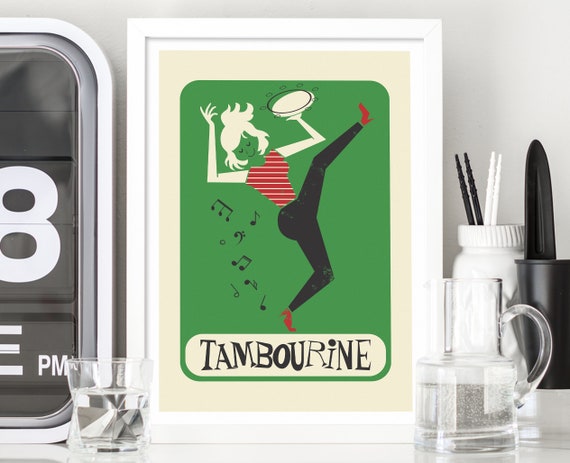The photograph showcases a collection of items centered around a vividly colorful, screen-printed piece of artwork. The main focus is a framed picture of a woman energetically dancing, one leg kicked high, accompanied by musical notes suggesting she’s moving to music. Dressed in a red and white striped shirt, black pants, and red shoes, she holds a tambourine. Her arms, hair, and tambourine are rendered in white, standing out starkly against the solid olive-green background. Below the woman, the word "tambourine" is prominently displayed in a blocky, black-and-white font. Surrounding this vibrant image are various monochromatic objects: to the right, two cups with what appears to be chopsticks or brushes, and a partial view of a clock showing the number 8 and "PM." To the left, there’s a clear glass mug with liquid, a smaller glass with liquid, and an assortment of black-and-white items including a flask with grainy black powder and a shot glass with a quartz crystal base. These surrounding elements are arranged in such a way that they accentuate and bring attention back to the central, lively artwork of the dancing woman.